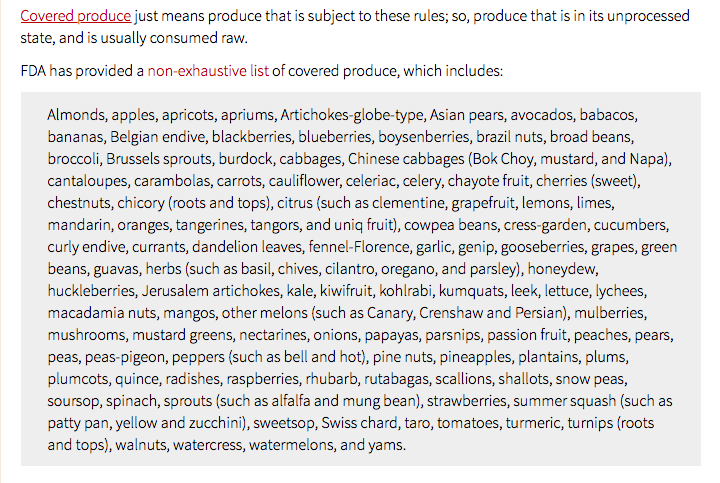The screenshot features a section of a website, with a layout that includes a vertical, tan-colored line on the left-hand side. The background of the page is primarily white, while the main body contains text inside a gray box. Above this gray box, the text "covered produce" is underlined in red. This section states, "covered produce" refers to produce that is subject to specific regulations; produce that is in its unprocessed state and is usually consumed raw. The text continues with an explanation that the FDA has provided a non-exclusive list of covered produce, with "non-exclusive" also highlighted in red. This list includes a variety of items such as almonds, apples, apricots, artichokes (short globe type), Asian pears, avocados, Babaco, bananas, Belgian endive, blackberries, blueberries, boysenberries, Brazil nuts, and roasted beans. The list spans over several lines, potentially comprising a dozen to a dozen and a half items, before continuing with more produce items.